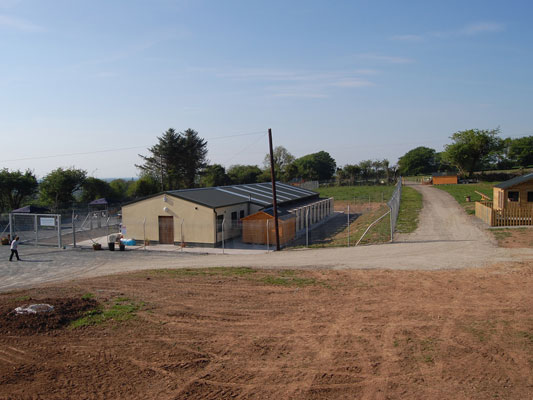The outdoor daytime photograph showcases a rural scene with a prominent one-story building near the center and slightly left. The structure resembles a storage facility or perhaps an animal kennel, complete with light tan walls and a central rectangular door. The roof is slightly pitched and gray, possibly with solar panels though not explicitly clear. Enclosing the space, a large chain-link fence extends on the left side, with additional fencing visible on the right. The setting appears well-secured, likely more functional than residential.

In the immediate foreground, a dirt patch dominates, marked by numerous tire tracks indicating frequent vehicle activity. This connects to a gravel road that runs horizontally in front of the building and extends into the background to the right. Adjacent to this road, on the leftmost part of the image, a person can be seen walking on the pavement, adding a human element to the otherwise still scene.

Further right, stalls or smaller structures are visible, possibly part of the same facility or an adjacent one. Another perpendicular street intersects near these structures, leading to a smaller shed with a wooden fence around it.

The background is a picturesque collection of fully grown green trees under a deep blue sky, dotted with wispy white clouds, adding a touch of serenity to the otherwise utilitarian landscape. The image is brightly lit and sharply focused, bringing out the details of this rural tableau.